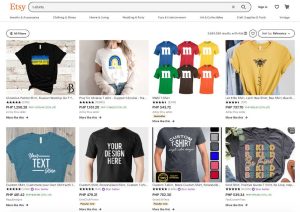The image appears to be a screenshot from an Etsy page, albeit a very small one that makes the details somewhat difficult to discern. At the top of the page, there's a search bar designed for users to refine their search queries. Below the search bar, several drop-down menus are visible, likely providing options to filter search results by categories, price range, and other criteria.

The main focus of the image is a display of various t-shirts, each with a distinct design and color. There are eight images in two rows. Starting with the top row:
1. A black t-shirt with an unspecified design.
2. A young woman modeling a white t-shirt with a colorful, though unclear, graphic print.
3. A collection of six t-shirts in the classic M&M colors, each featuring a prominent "M" logo—representing the colors of the iconic candy.
4. A yellow t-shirt adorned with a bumblebee and some additional decorative elements.

Moving to the second row:
1. A teal-colored t-shirt with the word "text" visible in the center.
2. A black t-shirt modeled by a gentleman, featuring the phrase "Your Design Here".
3. Another gentleman modeling a t-shirt; details of the design are unclear.
4. A plain gray t-shirt without any visible design.

Each t-shirt showcases diverse styles and graphics, highlighting the variety of customizable apparel available on Etsy.